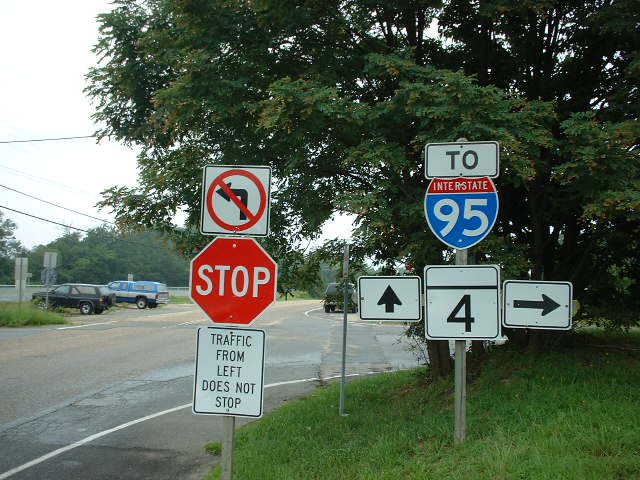The image is a vibrant outdoor photograph capturing a bustling intersection. In the foreground, a collection of street signs dominates the scene. The most prominent sign is an octagonal red stop sign with bold, white letters. Directly below this, a rectangular white sign with a black border declares in all capital letters, "TRAFFIC FROM LEFT DOES NOT STOP."

Further to the right, another sign showcases the numbers "Interstate 2" and "Interstate 95." Below this, a metal post features a directional sign with the number four, accompanied by black arrows pointing straight ahead and to the right.

In the midground, a grand tree with an abundant canopy of green leaves stretches out, adding a touch of nature to the urban setting. Directly behind the tree, a roadway extends into the scene. A car actively drives down this road, while on the side, an older model Suburban, painted in blue and white, is parked beside a sleek, black SUV.

This detailed composition captures a moment of everyday traffic amidst a mix of natural and urban elements, blending movement and stillness in the same frame.